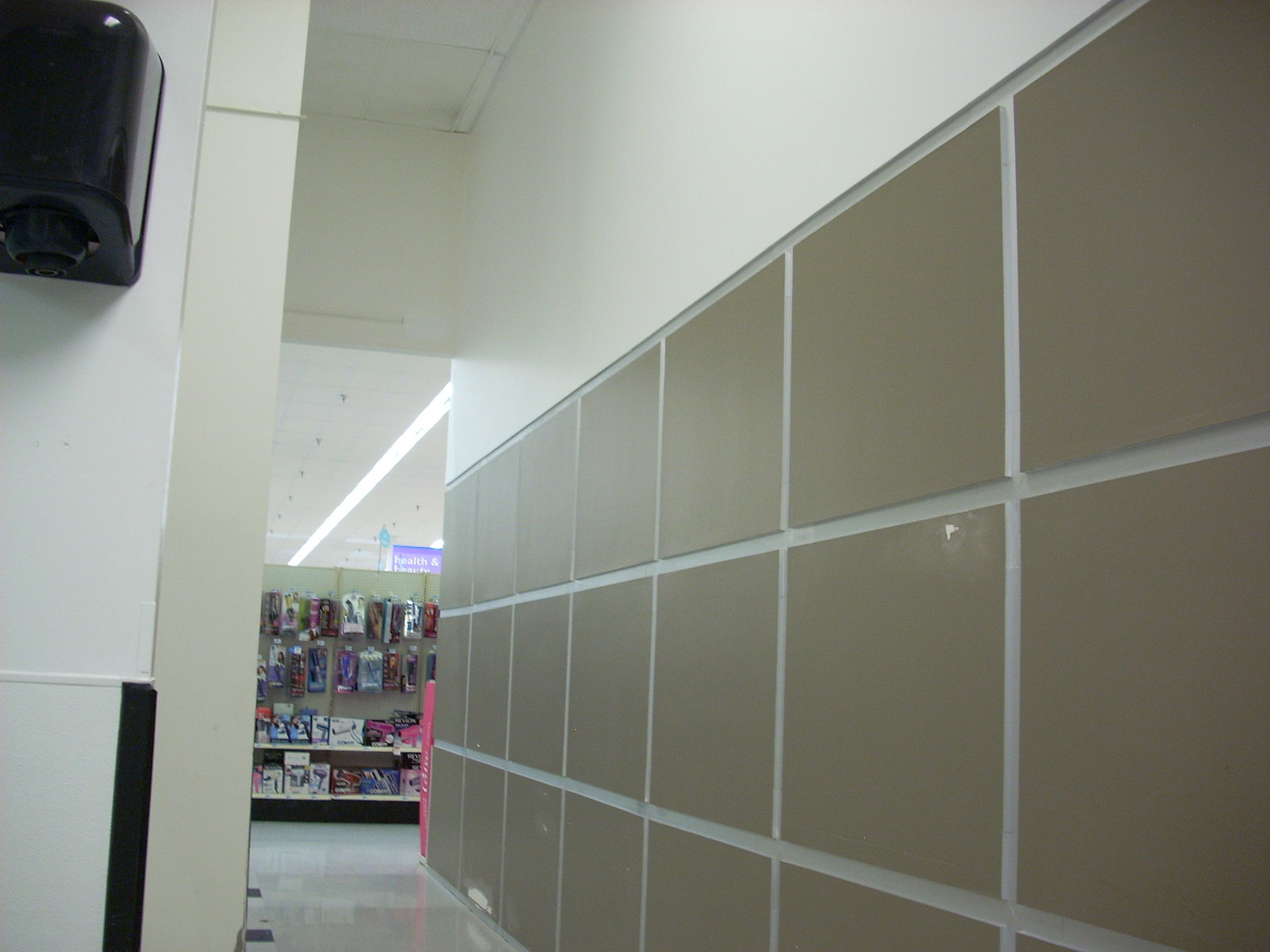The color photograph depicts the interior of a department store, specifically focusing on the hallway leading out from a bathroom area. On the left side of the hallway, part of a black hand dryer is visible, attached to a wall covered with large white tiles. The adjacent section of the wall transitions into brown tiles with a solid white surface above them. To the right of the hallway is an arrangement of cubbies or storage squares, which are brown with white borders, organized into three vertical rows stacked with seven squares each, although currently empty.

Ahead in the hallway, one can see into the main area of the department store where various items, such as clothing and other goods, are displayed on hangers and shelves. Prominently featured are two white shelves holding products like hair dryers in assorted colors—red, pink, white, and blue—and potentially hair straighteners. There is a pink item, approximately two feet tall, standing on the floor among other items for sale, garnishing the end of the aisle. The ceiling in the image is plain white, contributing to the overall clean and orderly appearance of the scene.